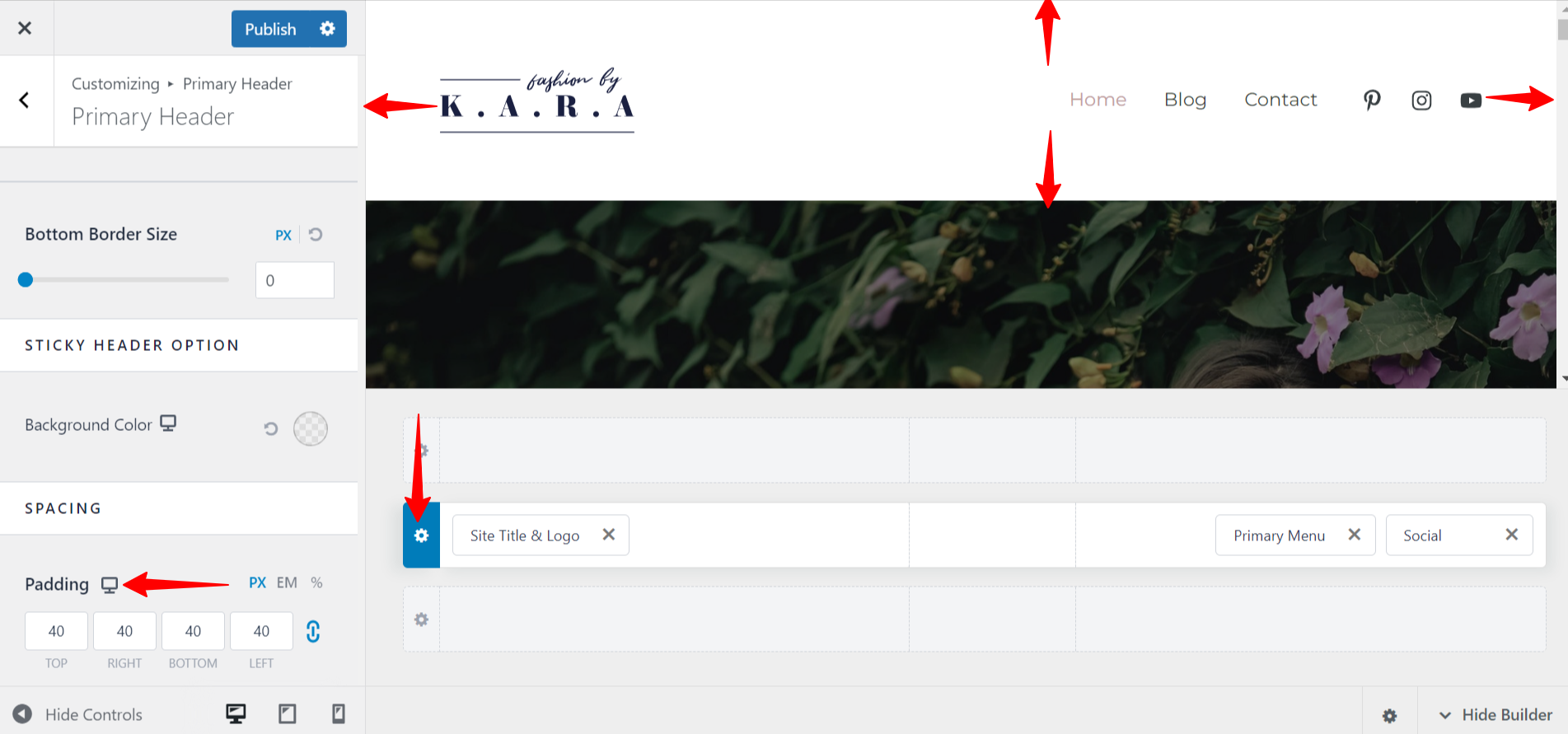The image is a screenshot of a webpage from a site titled "Fashion by K.A.R.A." The logo "Fashion" is written in delicate cursive script, while "K.A.R.A." is presented with each letter capitalized and separated by periods (K.A.R.A.). The webpage features six red arrows indicating various sections. 

1. A red arrow points left at the primary header where "Fashion by K.A.R.A." is displayed.
2. Two arrows, one pointing up and the other down, indicate the "Home" section located at the top center of the page.
3. Another arrow points right at a play button, resembling a YouTube icon.
4. A downward-pointing red arrow highlights a blue gear icon representing settings.
5. An arrow is positioned next to the word "Padding," which is accompanied by a TV icon.
6. The last arrow points left to the area marked "PX."

Each arrow denotes significant segments of the webpage, guiding the viewer's attention to specific interactive elements and settings.